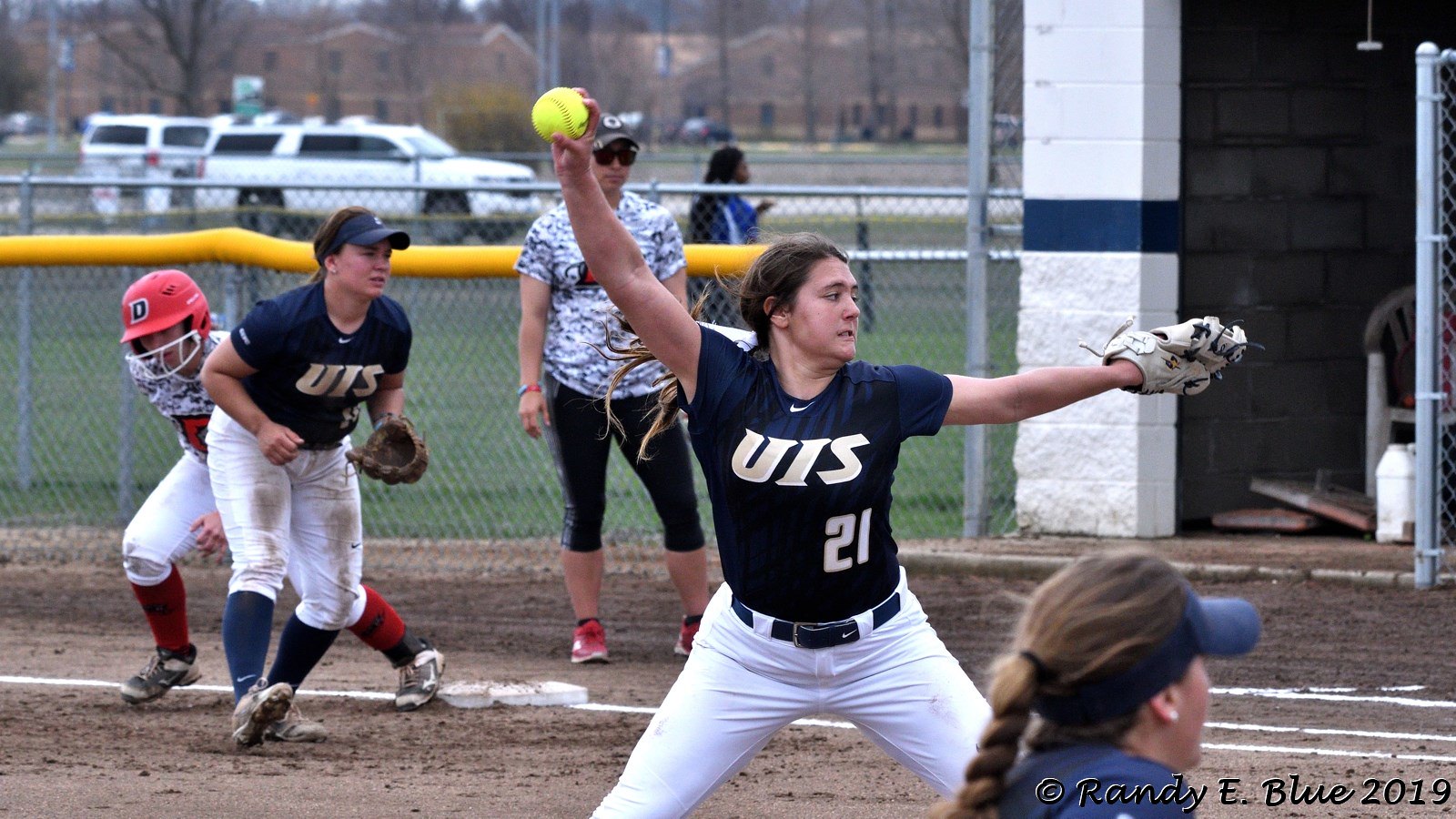This photo captures an intense moment in a female softball game, centered on the right-handed pitcher, number 21, from team UIS. Donning a dark blue jersey with 'UIS' emblazoned on the front, white pants, and a white mitt, she is poised to deliver a pitch with a bright yellow softball in her hand. Her brown hair is pulled back and her stance is wide, exuding focus and energy. To her left, on what appears to be the first base, a teammate in a dirty uniform and gloves is ready for action. Nearby, an opposing team's player sporting a red helmet waits intently while a coach with a blue visor stands behind the base. The game is set outdoors on a muddy, grass-bordered field, adding to the rugged ambiance. The scene is captured with the inscription "Randy E. Blue, 2019" at the bottom right corner, indicating the photograph's origin.